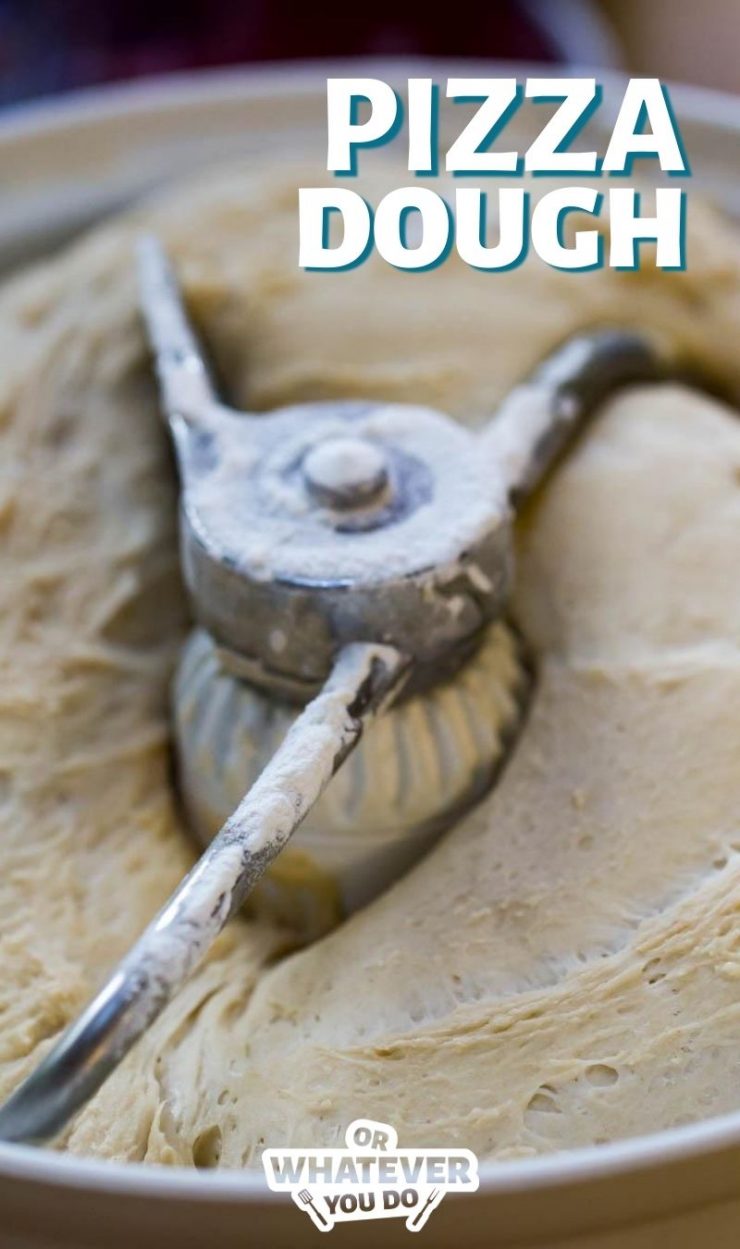This image features an extreme close-up of a pizza dough mixer. Dominating the center is a large, metallic mixing arm set inside a bowl filled with light brown pizza dough. The machine appears industrial with a white base and metal components, including two metal rods, giving a robust impression. Toward the top right, in white text with a subtle blue shadow, the words "pizza dough" are prominently displayed. The background at the top is slightly blurred, providing no significant detail and emphasizing the mixer. At the very bottom center, in a light tan text with a white border, the phrase "or whatever you do" is visible. Accompanying this text are small icons: a spatula on the left and a two-pronged steak fork on the right. The overall composition suggests an advertisement with a focus on the functionality and utility of the mixer within a possibly professional setting. The background colors blend from maroon to brown, complementing the prominent hues of blue, white, and tan in the text and border.